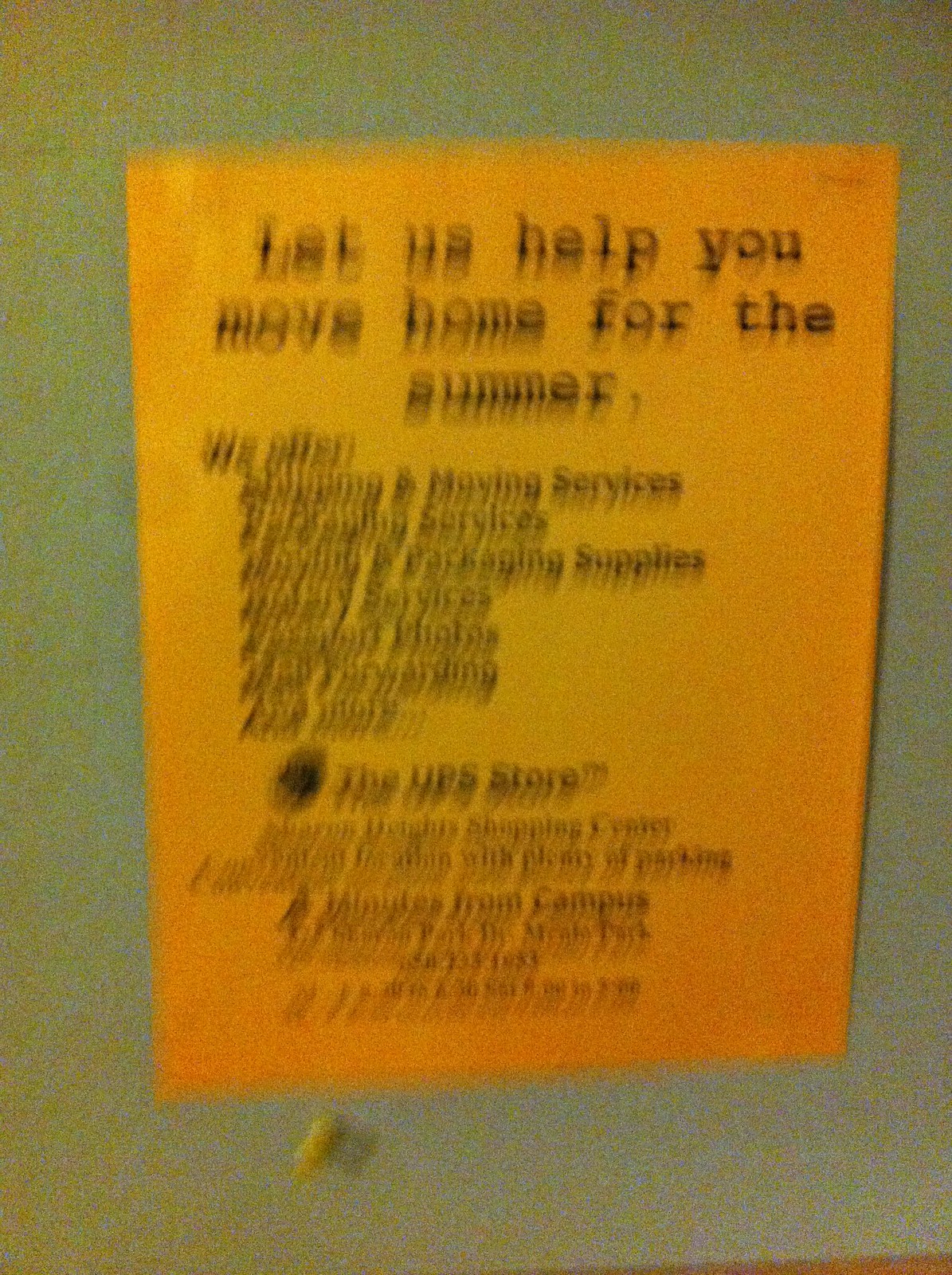This is a very blurry, low-quality photograph of a deep golden-yellow-orange piece of paper stapled to an off-white wall with a yellow pushpin at the bottom. The paper, featuring black block-letter text, has a slightly shadowed space behind it, indicating it isn't fully flush with the wall. Due to the blurriness, much of the text is difficult to decipher, but the visible portion reads, "Let us help you move home for the summer. We offer shipping and moving services." There's additional text that is largely unreadable. Towards the bottom of the paper, "The UPS Store" is clearly visible, along with indications of a phone number and other blurred details, giving a double-vision effect. The background of the image is somewhat splotchy, combining white and yellowish tones.